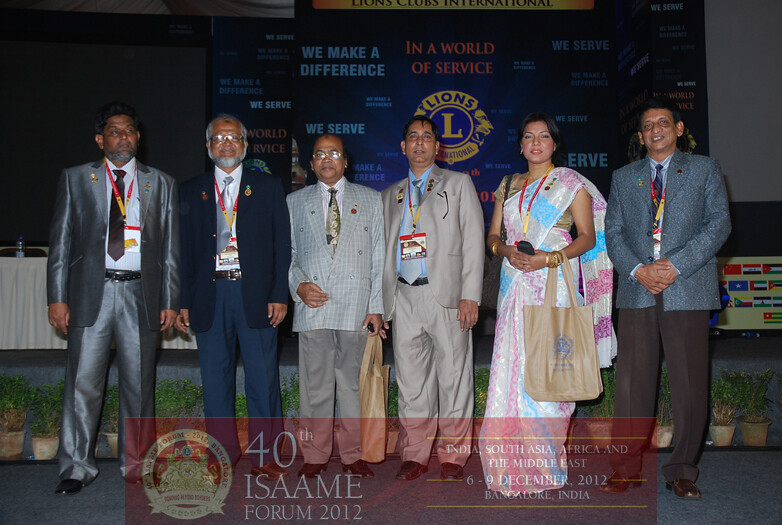Captured in this image are six individuals standing in a line, partaking in what appears to be either a wedding ceremony or another formal event. All of the men are dressed in elegant suits, while one woman is adorned in a traditional Indian dress. They are all facing the camera, exuding a sense of solemnity and occasion. Behind them, there’s a dark blue backdrop prominently featuring the Lions logo, along with multiple other logos and flags that contribute to a formal ambiance. At the bottom of the screen, the text "40th Stomie Forum 2012" along with its corresponding logo is displayed. Flanking the group are small potted plants, adding a touch of greenery to the solemn setting.